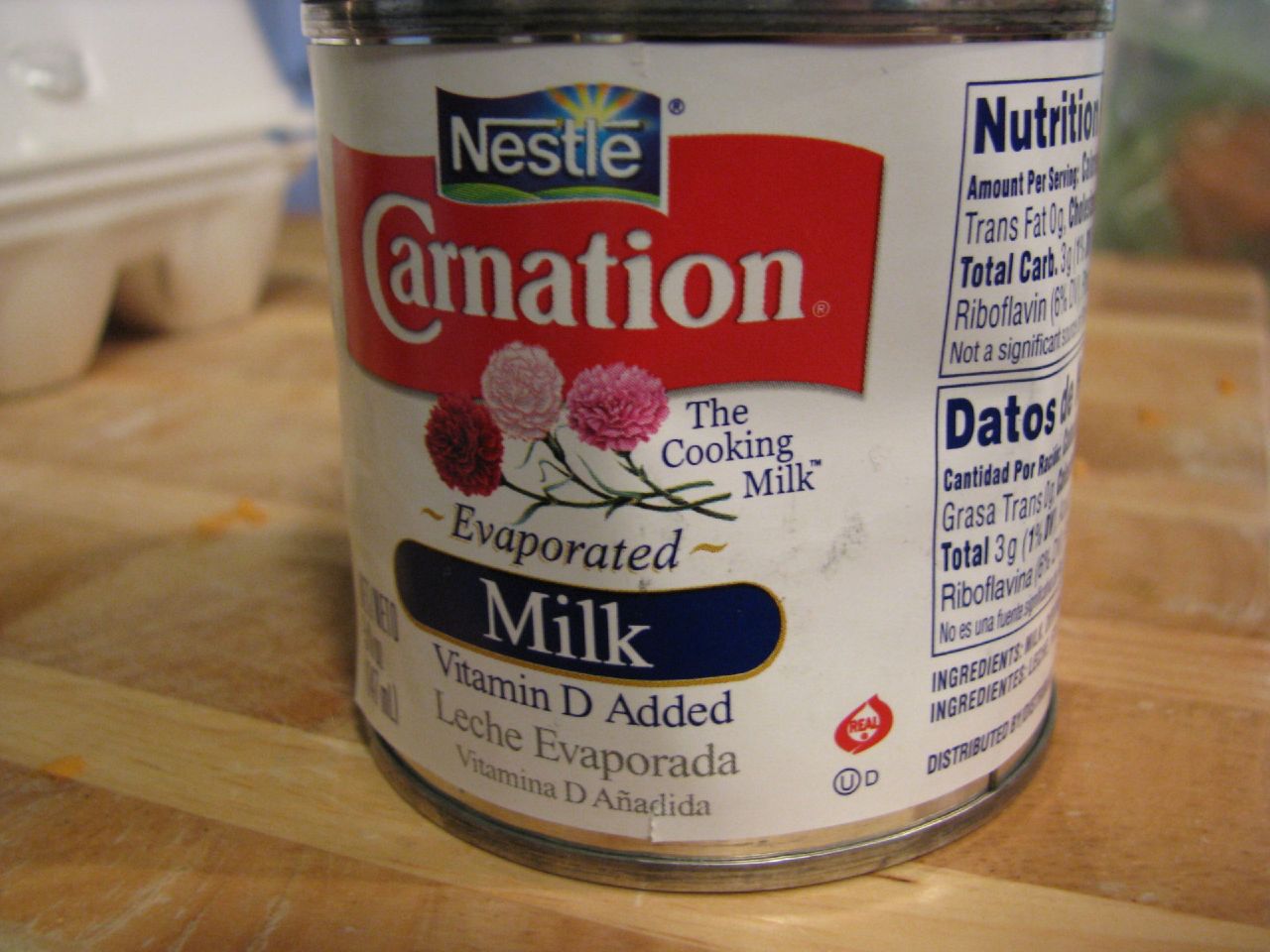The close-up color photograph showcases a slightly dented tin of Nestle Carnation Evaporated Milk positioned on a light beige wooden surface, which could be a kitchen worktop or a chopping board. The label prominently features the Nestle logo in a blue banner at the top, followed by the Carnation brand name in a red banner. Below this, three Carnation flowers are illustrated: one light pink, one vibrant pink, and one dark red-purple. Additional text on the label indicates that the product is the "cooking milk" and has added Vitamin D. Orange shavings, possibly carrot, are scattered around the tin, suggesting recent kitchen activity. In the left background, a blurred white carton of eggs is visible, though only partially showing two egg cup shapes, hinting its position from the hinged side. The top of the tin is slightly cropped out of the frame, emphasizing the close-cropped nature of the photograph.